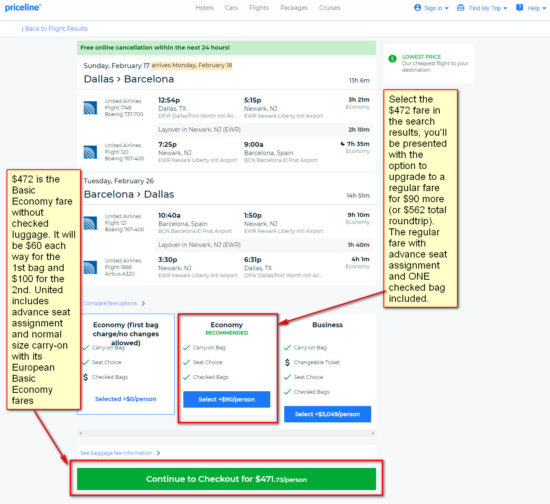The image showcases a website page from Priceline, identified by its logo in the top left corner. Across the top menu bar, a series of headings can be seen, including 'Hotels,' 'Cars,' 'Flights,' 'Packages,' and 'Cruises.' On the right-hand side of the header are options for 'Sign In,' 'Find My Trip,' and 'Help,' highlighted in blue.

The main content of the screen reveals details of a booked round trip from Dallas to Barcelona, scheduled for February. Various selection boxes are visible, allowing users to choose their trip preferences, such as economy or business class. One such box, corresponding to economy class, is enclosed in a red rectangle. An annotation box, colored yellow with a red border, points to this economy box and contains the following text: "Select the $472 fare in the search results. You'll be presented with the option to upgrade to a regular fare for $90 more. The regular fare includes advanced seat assignment and one checked bag."

At the bottom of the screen, a green button is also highlighted with a red box and an arrow pointing to it. A yellow annotation box with red borders next to this green button contains additional explanatory text: "$472 is the basic economy fare without checked luggage. It will be $60 each way for the first bag and $100 for the second. United includes advanced seat assignment and normal size carry-on with its European basic economy fares."